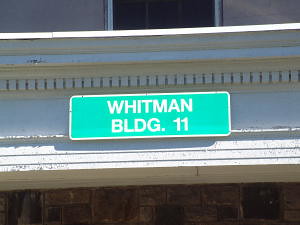A small, square image showcases a portion of an old building facade. At the center of the image is a green sign with white lettering that reads "Whitman BLDG 11." The building itself appears worn, with patches of white paint peeling to reveal the underlying surface. At the top of the image, part of a window opening is visible, hinting at the structure's residential or commercial use. The bottom section of the facade reveals a layer of brickwork, further emphasizing the building's aged and weathered appearance.